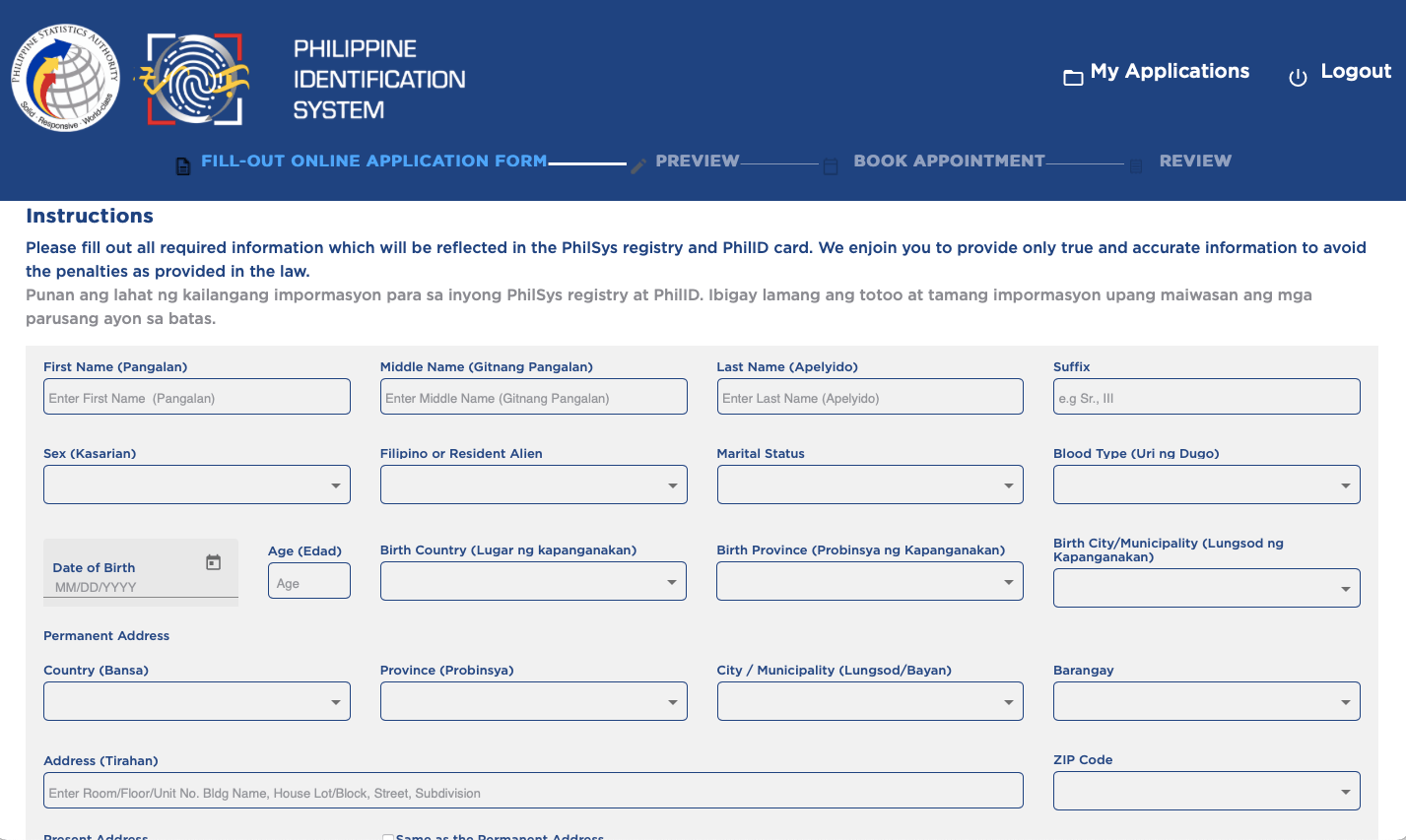The image illustrates a webpage that displays the Philippine Identification System online application form. Prominent elements include a "My Applications" button and a "Logout" button on the top right corner, emphasizing user accessibility and security. The interface is structured like a form and is divided into multiple steps, with the current view focusing on Step 1 of 4. Subsequent steps include 'Preview,' 'Book Appointment,' and 'Review,' guiding the applicant through a systematic registration process.

At the beginning of the form, there's a section titled "Instructions," advising applicants to provide true and accurate information, as inaccuracies could lead to legal penalties. The form requests various personal details, each accompanied by a corresponding Filipino translation for inclusivity. Required information includes:

- First Name
- Middle Name
- Last Name
- Suffix
- Sex
- Citizenship Status (Filipino or Resident Alien)
- Marital Status
- Blood Type
- Date of Birth
- Age
- Country of Birth
- Province of Birth
- City of Birth
- Permanent Address Information, including Country, Province, City, and Barangay (a Filipino term for district or neighborhood)
- Zip Code

Numerous fields are presented as drop-down boxes for streamlined data entry. The page's design and bilingual instructions indicate that it serves as the official platform for registering in the national ID system governed by the Philippine government.